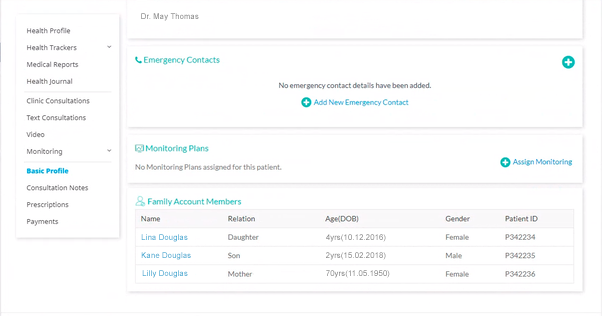Screenshot of a Health Management Website

This image is a screenshot of a health management website, presumed to be related to Dr. May Thomas as indicated by the prominent display of her name at the top of the page. The interface appears to be designed for scheduling medical appointments and managing personal health information. The layout includes several navigation sections located on the left side of the screen, listing options such as Health Profile, Health Trackers, Medical Reports, Health Journal, Clinic Consultations, Text Consultations, Video, and Monitoring. Both Health Trackers and Monitoring have drop-down menus, suggesting further sub-categories.

Beneath these main sections, additional options are visible, including Basic Profile, Consultation Notes, Prescriptions, and Payments. 

Central to the page, there is a segment dedicated to Emergency Contacts, highlighted by bright green text and a phone icon on the top left. Adjacent to this, on the top right, there is a green circular button with a plus symbol, indicating the functionality to add new contacts. Below this header, a message reads, “No emergency contact details have been added,” along with a prompt to add emergency contact information.

Although the image is somewhat blurry and small, it is clear that the website serves as a comprehensive tool for patients to manage their healthcare appointments, records, and emergency contact details.